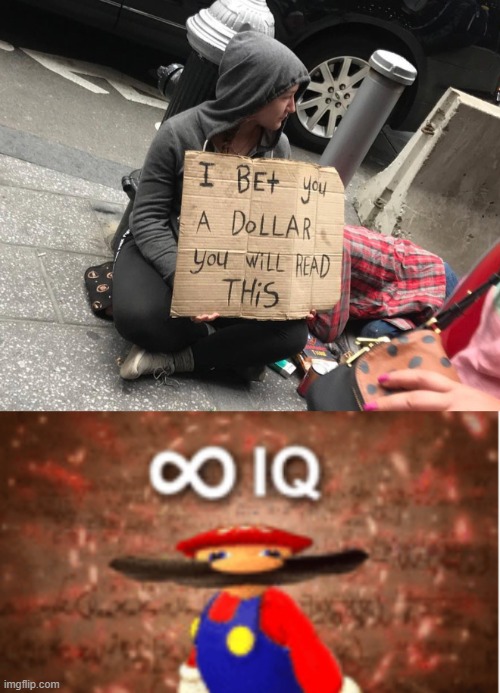The caption is split into two parts to describe two distinct images.

**Top Image**: A woman dressed in a grey hoodie with the hood up, black tights, and grey shoes with white soles is sitting on a sidewalk, leaning against a fire hydrant with a black pillow top. She has a purse in front of her and is holding a cardboard sign that reads, "I bet you a dollar that you will read this." To her right, there is a sleeping bag, several items including what appears to be cigarettes, and a book. She gazes off to the side as a person carrying a purse walks past. In the background, a car is visible.

**Bottom Image**: A distorted image of Mario from Super Mario 64 features his head squished and mustache extended. He is dressed in normal attire with blue overalls, big gold buttons, a red shirt, and white gloves. Above him, a sideways 8 symbol, representing infinity, suggests "infinite IQ."